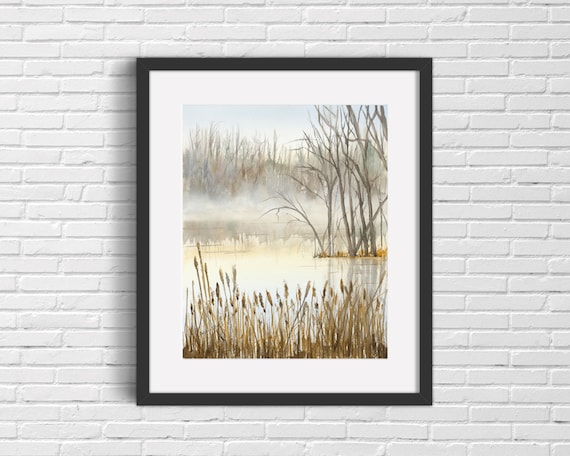A striking painting is mounted centrally on a stark white brick wall, which occupies the majority of the viewable area, leaving about six inches of wall space on either side. The artwork is framed in a sleek black frame with a white matte, creating a distinct contrast against the textured backdrop. The painting depicts a hauntingly beautiful marsh on a foggy day, dominated by a row of delicate pussy willows in the foreground. Beyond the willows, a misty lake spreads out, its surface partially obscured by thick banks of fog. On the left-hand side of the painting, bare branches of trees jut out, adding to the eerie atmosphere. A backdrop of high grasses and more pussy willows emerges through the veil of fog, their faint reflection shimmering on the lake's shadowed waters. The entire scene evokes a sense of tranquility and mystery, despite the absence of a visible signature on the artwork.